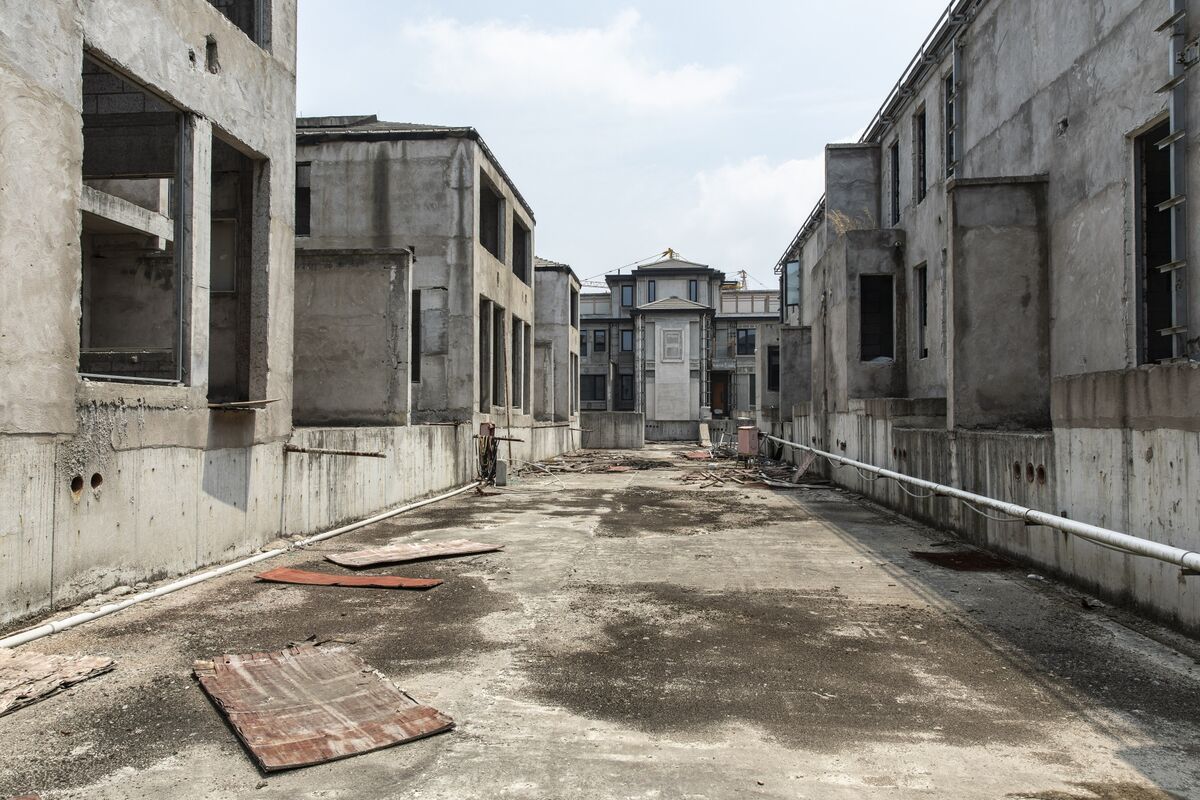The image features an eerie, abandoned urban scene marked by desolation and decay. A concrete path stretches through the center, flanked by derelict three-story cement buildings riddled with gaping window openings. On the left, two buildings are separated by a small wall, their facades punctuated by dark water stains. A few pieces of red and brown cardboard or material are scattered along the path. On the right, a long building with protrusions displays similar signs of neglect, albeit in slightly better condition. Most centrally positioned is a partially intact three-story building with some windows still in place and a middle tower crowned with triangular roofs. In the far background, a more intact building with white paneling and green features stands, possibly still inhabited or functional, contrasting starkly with its surroundings. The sky above is a mix of light blue and white, dotted with two white clouds, casting a faintly surreal light over the silent, war-torn landscape.